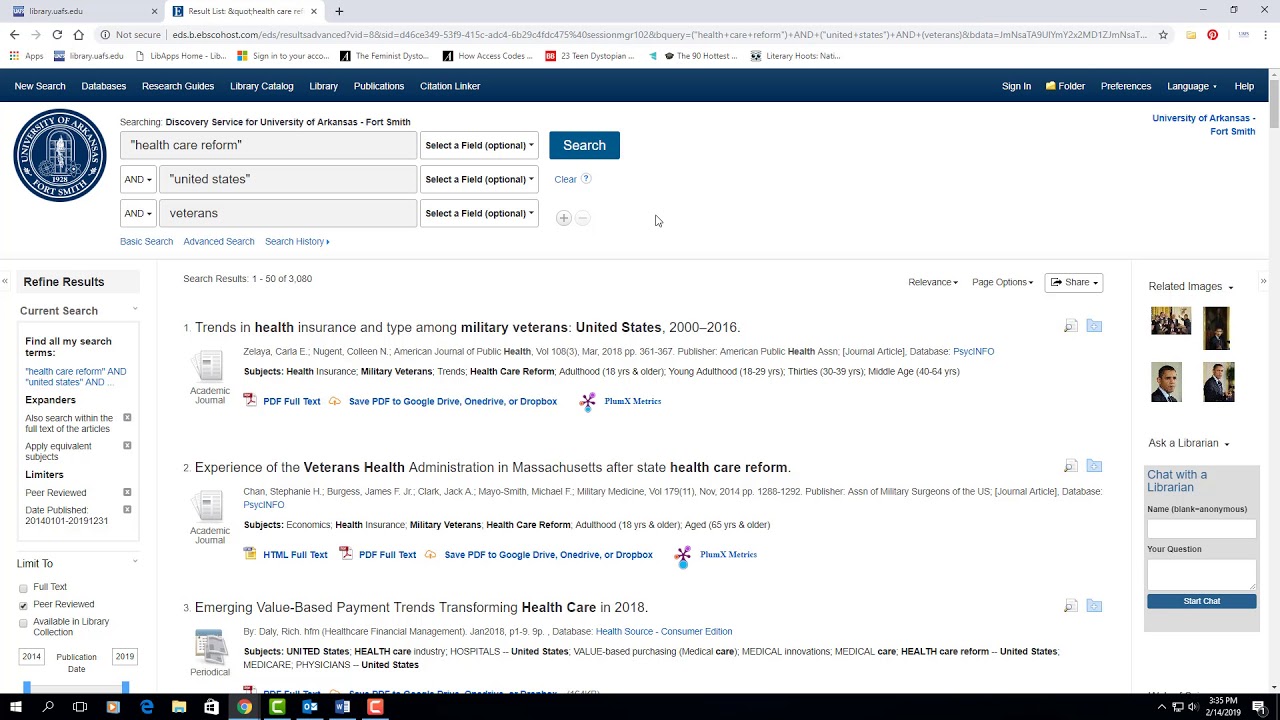This screenshot captures a University of Arkansas Fort Smith web page on a desktop browser. The browser has two tabs open: the first tab labeled "library.uofa.edu" and the second tab labeled "results list, care reform," with the latter being the current view as indicated by its highlighted state. 

Below the tabs, the browser interface includes a search bar and favorites icons. The webpage itself features a dark blue header with navigation links including "New Search," "Databases," "Research Guides," "Library Catalog," "Library Publications," and "Citation Linker" on the left, and "Sign-In," "Folder," "Preferences," "Language," and "Help" on the right. 

The main body of the page has a white background, starting with a large circular logo for the University of Arkansas Fort Smith in the top-left corner. Next to the logo, text boxes and dropdown menus are available under the heading "Searching Discovery Services for University of Arkansas Fort Smith." 

The search interface consists of several rows of search fields:
- The first row includes a large text box containing the term "health care reform," followed by a dropdown menu labeled "Select a Field (optional)."
- The second row has a dropdown menu set to "and," a text box with "the United States" in parentheses, and another dropdown menu labeled "Select a Field (optional)."
- The third row mirrors the structure of the second, with "and" in the dropdown menu, a text box containing "veterans," and another "Select a Field (optional)" dropdown menu.

There is also a prominent blue "Search" button on the top right. Below this search section, the webpage displays search results in the center. To the left of the results, a thin vertical panel titled "Refine Results" offers various filters for narrowing the search, with a "Current Search" section listing clickable options to limit the search scope.